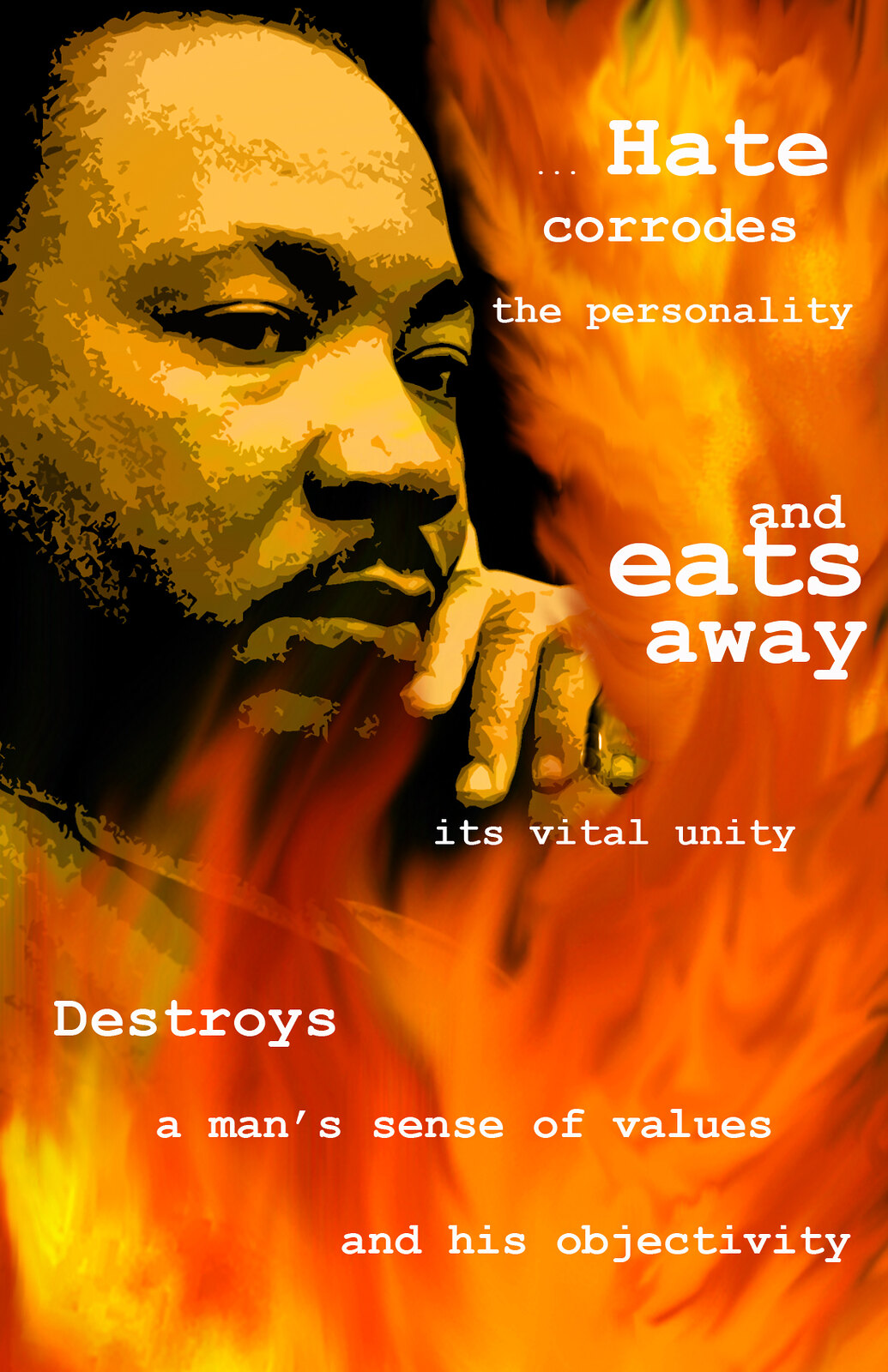This rectangular, color movie poster depicts a serious tone, featuring a digitally painted image of Martin Luther King Jr. The background is dominated by fiery hues of orange and yellow, resembling flames, which emphasize the intense theme of the poster. King's face is prominently displayed on the left side, showing him in a contemplative and somewhat somber pose, with his fingers resting below his lips and along his cheek, highlighting his thoughtful expression. His hairline is receding, and he has a distinct mustache. The body cuts off into the flaming background, leaving the focus on his face and hand.

Overlaying the right side of the poster is an impactful quote in varied sizes of white text. The larger words emphasize the gravity of the message. At the top, it reads, "Hate corrodes the personality," continues in smaller letters, "and eats away its vital unity," and concludes at the bottom with, "destroys a man's sense of values and his objectivity." The text arrangement and the intense color scheme work together to underscore the powerful message of the advertisement.